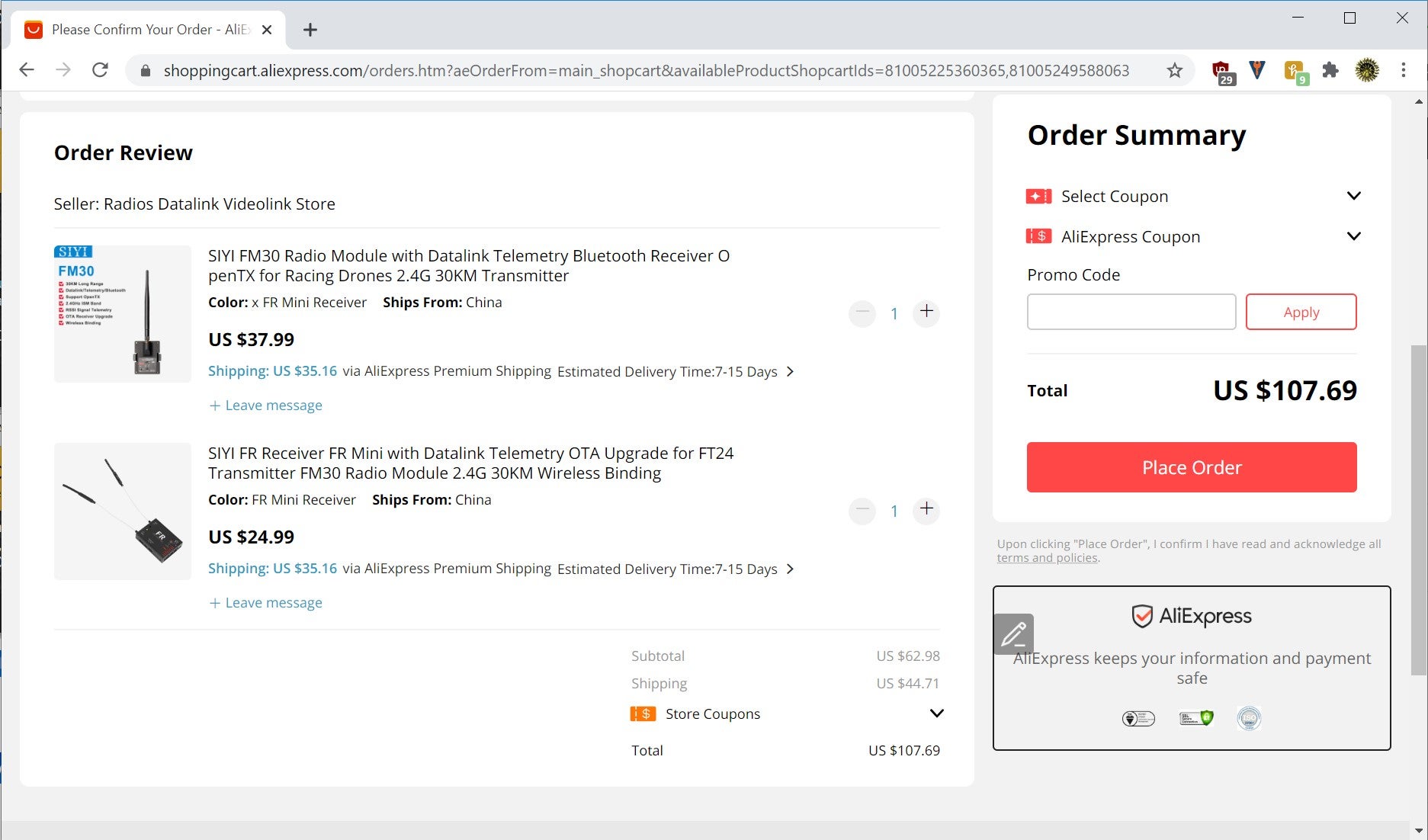The image is a detailed screenshot from the AliExpress website, showing an order summary and review section for a purchase. At the top of the browser, a long URL is visible, and in the top-right section, there are several icons such as a puzzle piece and a gear, though their exact functions are unclear. The order summary section indicates the purchase of two items: a "SIYI FM-30 Radio Module with Data Link Telemetry and Bluetooth Receiver" and a "PEN-TX for Racing Drones." The image features a picture of the radio module on the left, priced at US $37.99 with shipping costs of $35.16. Below it, the mini data link telemetry receiver is listed at $24.99, also with shipping priced at $35.16.

The subtotal for the items amounts to $62.98, with the total shipping cost being $44.17, resulting in an overall total of $107.69. The right side of the screenshot lists options for applying a select coupon, AliExpress coupon, and promo code, although these fields are empty. Prominently displayed is the total cost of $107.69, accompanied by a red "Place Order" button. Below the button, there is a shield icon suggesting that AliExpress ensures the safety of the buyer's payment and information. A scroll bar is visible on the right side of the browser, indicating that there is more content to scroll through.